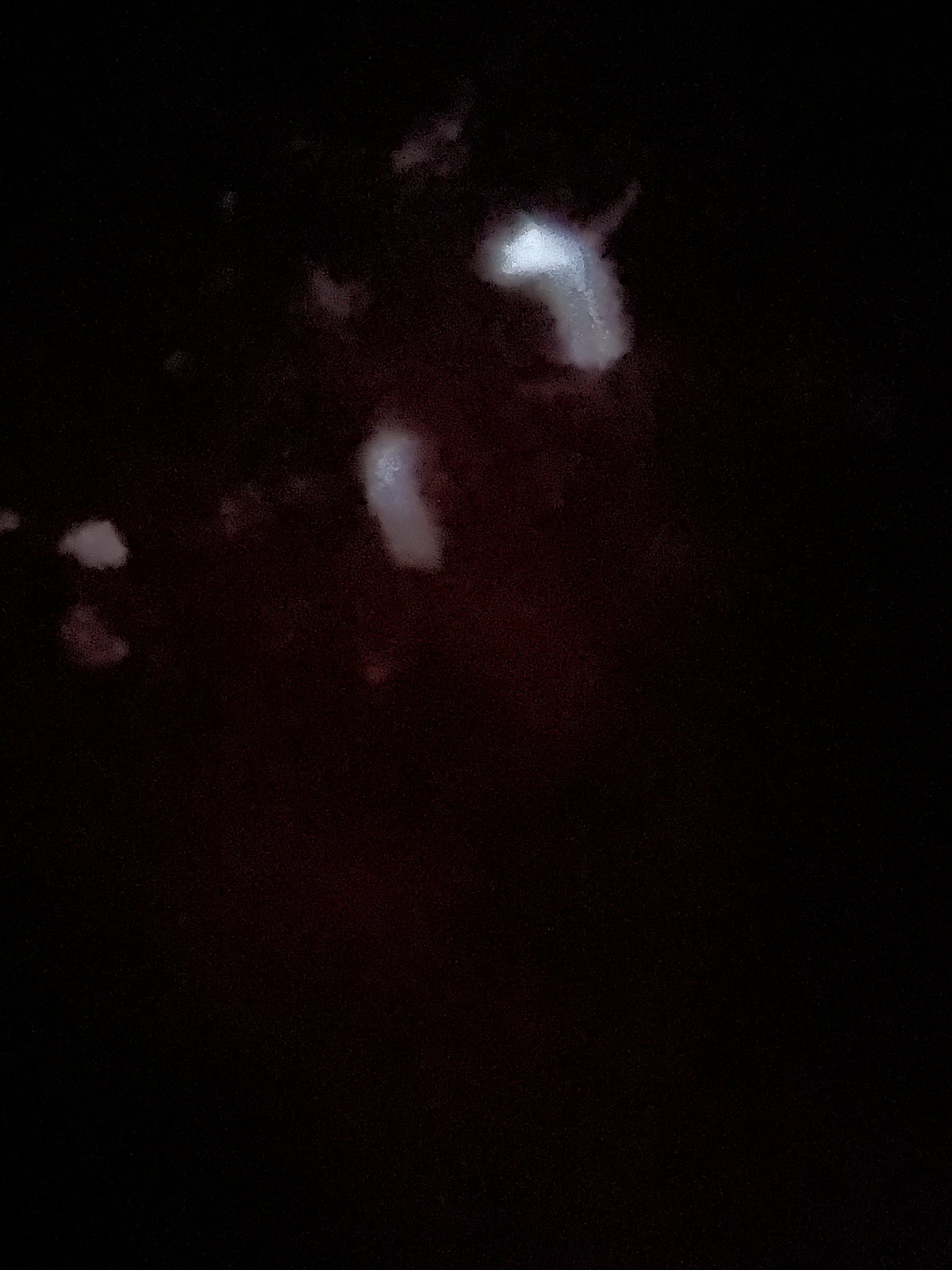This image presents an abstract, predominantly black background with a faint central red glow, possibly indicative of a distant space explosion. The central red shape is accompanied by various white smudges and objects, resembling meteors or space debris emanating from the explosion. A notable white, blurry shape in the upper right of the center resembles a bent hand, covered by a sock with curved fingers. To the lower left of this, another white object, lighter and rectangular, curves at the top. On the left edge, slightly above center, a light gray triangle is visible. The composition has an abstract, art-like quality, with the majority of the image enveloped in darkness, highlighting the central red and scattered white elements against the black backdrop.